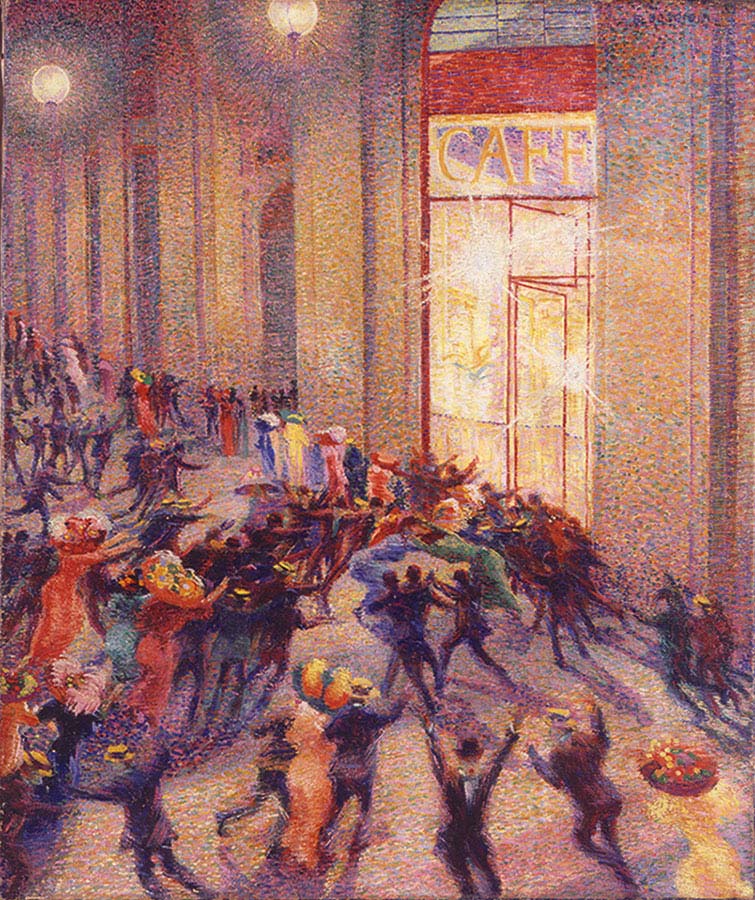This impressionistic painting depicts a chaotic scene outside a large café, likely from the 1800s in France. The café, marked by a tall arched window and a red glass door partially open, is prominently labeled "CAFE" in yellow letters. Globe-shaped lights, approximately 25 feet high, illuminate the building's orange, textured walls. The café's façade is primarily glass, with some areas appearing to show damage, possibly from objects being thrown by the crowd. The upper-middle-class crowd, filled with women in fancy bonnets and hats, is densely packed and appears to rush towards the building, some with arms raised. The people, painted in vibrant, undefined colors, become smaller, giving a sense of depth as they recede into the scene. The overall ambiance hints at a frenetic, possibly violent atmosphere, accentuated by the flashes of light reflecting off the café's glass.